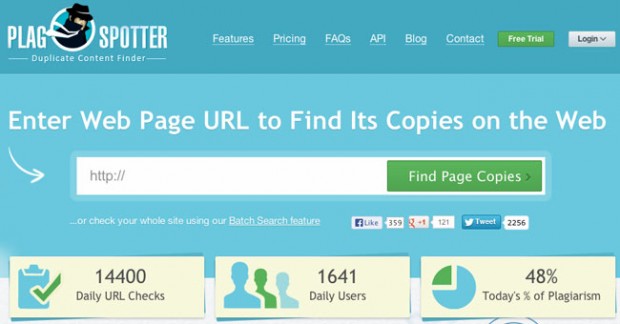The image depicts a website named "Plagg Spotter," designed with a dual blue background. At the top of the page, the website's name and logo are displayed prominently. On the left-hand side of the header, the logo features a man wearing a white tie and hat. The text "Plagg" appears in white, next to the logo, followed by "Spotter" also in white. Below the name, the phrase "Duplicate Content Finder" is written in small text.

Along the header, small white lettering lists the site’s sections: "Features," "Pricing," "FAQs," "API," "Blog," and "Contact." Towards the right side of the header, there are two buttons: a green "Free Trial" button and a white "Login" button.

Beneath the header, a lighter blue section invites users to "Enter web page URL to find its copies on the web" in large white letters. A small white arrow points to a search bar below the text. The search bar is white with a green "Find Page Copies" button on the right. Below the search bar, small text encourages users to "check your whole site using our batch search feature."

To the right of the search bar, social media icons display the site's popularity metrics: 359 Facebook likes, 121 Google Plus likes, and 2256 tweets.

Further down, three small rectangular windows provide additional data:

1. The first window displays "14,400 Daily URL Checks" accompanied by a clipboard icon with a checkmark.
2. The second window shows "1,641 Daily Users" next to three people icons.
3. The third window indicates "48% Today's Percentage of Plagiarism" with a pie chart icon.

The overall layout and design are aimed at emphasizing the website's functionality for finding duplicate content.